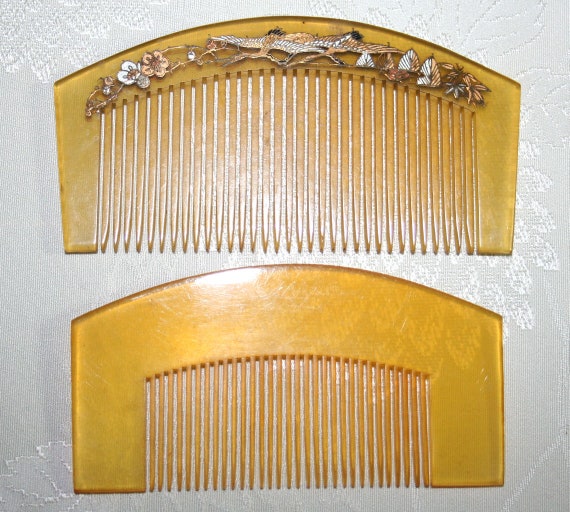The image features two antique hair combs designed for women, likely from the early 1900s, used to secure long hair. Both combs are of a light tan or yellowish-amber color, suggesting they are made from an early form of plastic, such as celluloid or bakelite. 

The larger comb, which has an arched shape, shows intricate decoration with stylized cranes, flowers, and leaves in bronze and silver tones, giving it an ornate and elegant appearance. This decorative element is set above the teeth of the comb. 

The second comb is smaller, thicker, and plain with no embellishments, presenting a simple utility in contrast to the decorative nature of the larger comb.

Both combs are placed on a plain piece of paper or background with no additional text or colors, emphasizing their vintage and possibly handmade quality. These combs would be ideal for anyone looking to recreate an authentic vintage hairstyle, capturing the essence of their era.